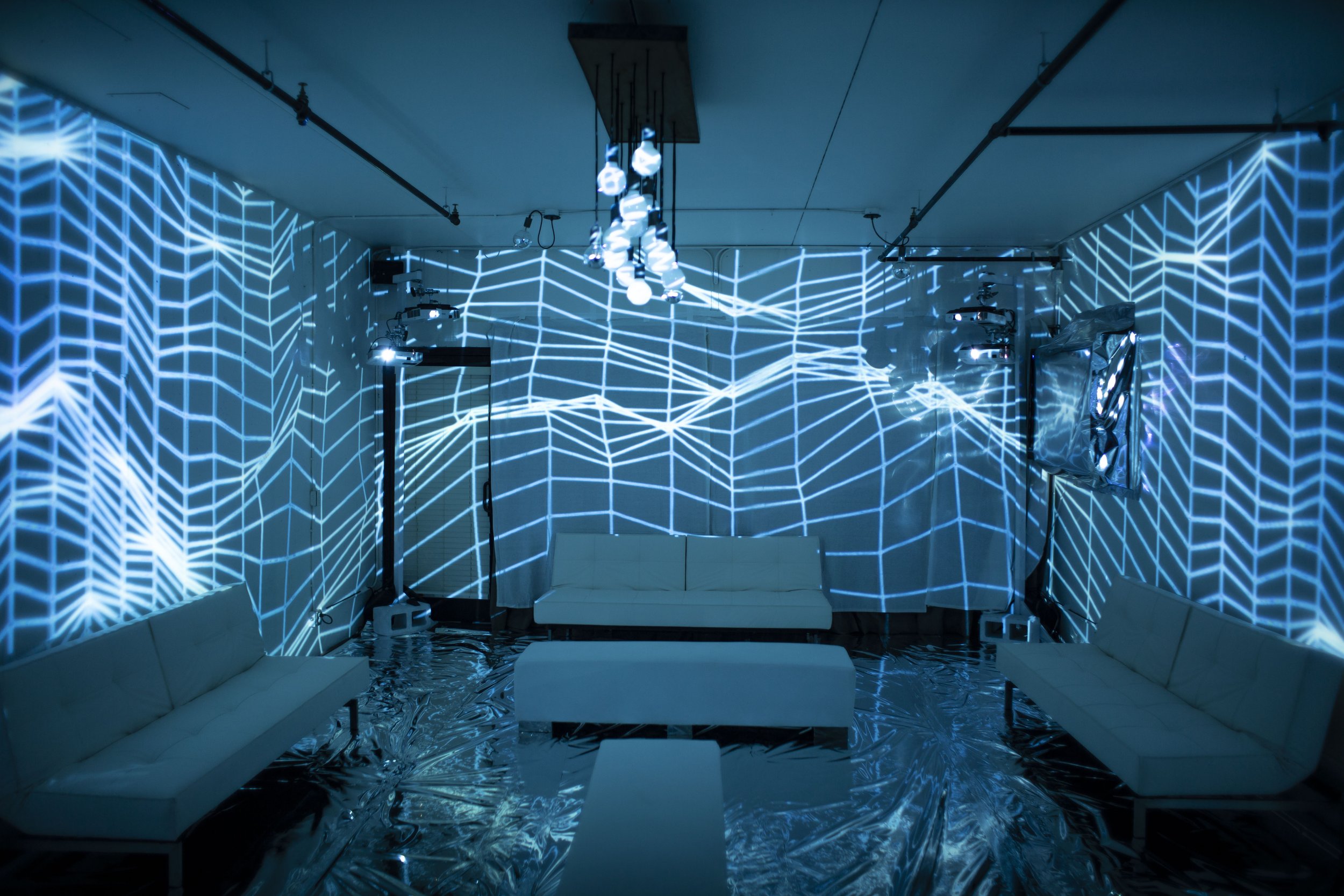This is an indoor image of a nightmarishly futuristic room with an unsettling color scheme dominated by shades of grey and blue. The room features three grey couches positioned against the walls, paired with a few matching ottomans or coffee tables. Overhead, a bundle of blue and white lights hangs from a dark ceiling, casting eerie shadows. The flooring appears to be covered in a shiny, crinkled material, possibly black plastic or reflective aluminum foil. The walls are bathed in an electric blue light, crisscrossed with white lines that resemble bending graph paper or electrical currents, heightening the room's surreal ambiance. Additional black pipes line the ceiling, but there are no people present in the image. Overall, the room's stark, high-tech vibe is both disconcerting and intriguing.